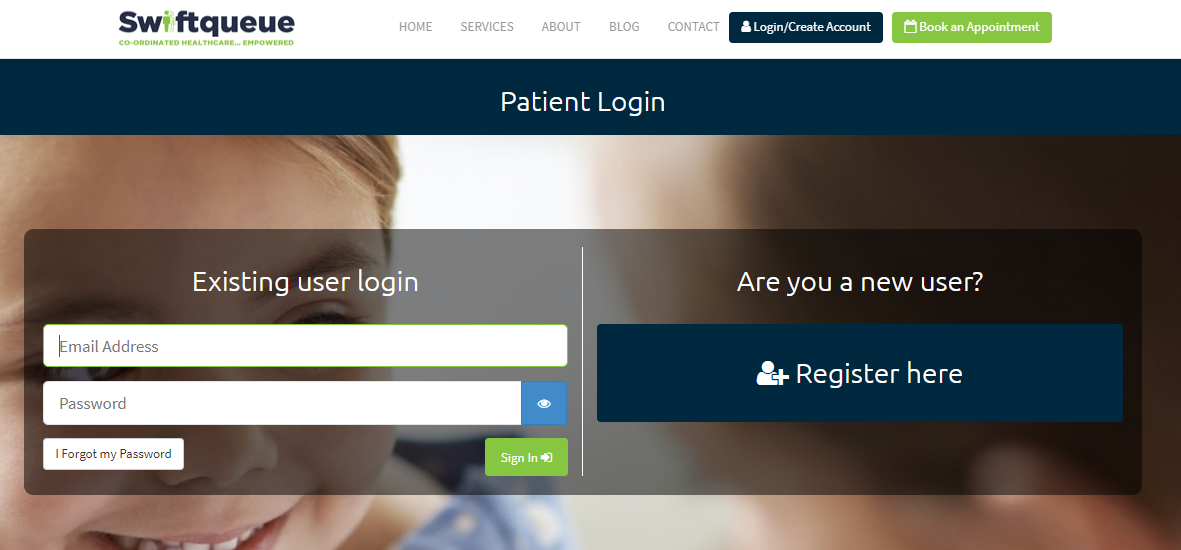The page features a long rectangular layout with the header prominently displaying "SWIFTQ" in blue and green letters. At the top center of the page are navigation tabs labeled HOME, SERVICES, ABOUT, BLOG, and CONTACT. On the top right, dark blue text reads LOGIN and CREATE ACCOUNT, while nearby in green text is BOOK AN APPOINTMENT.

Centrally located on the page is a bold, white PATIENT LOGIN header, directing users toward account access. Towards the bottom, there's an EXISTING USER LOGIN section where users can input their email address and password, with options to state "I Forgot my Password" and press a SIGN IN button. Additionally, on the lower right, it prompts "Are you a new user?" with an invitation to register.

The page employs a blue and white color scheme and includes images. Notably, there is a picture of a young child with blonde hair, olive skin, bright smile, and large wide eyes set against a pristine white background.